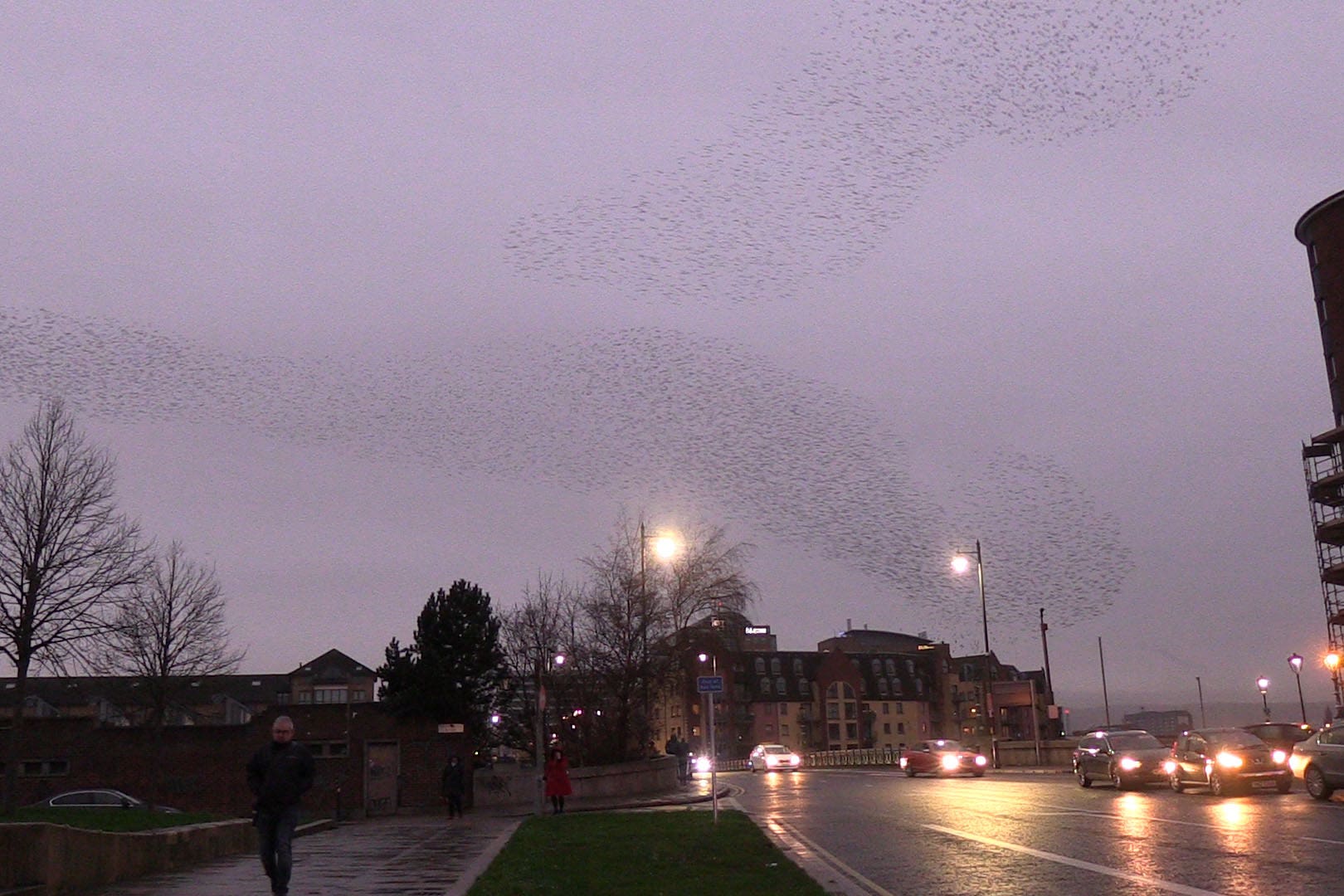This photograph captures a dynamic urban scene at dusk, characterized by a dramatic sky and busy street life. The sky, a light to medium gray with a purplish hue, is dominated by two massive flocks of birds, appearing as dark dots scattered across the expanse. The urban setting features industrial-looking multi-story buildings and office spaces in the background, giving an architectural depth to the scene. 

A wet, reflective roadway runs through the image, which is lined by glowing headlights from a line of vehicles traveling towards the right. A patch of green grass serves as a median, separating this bustling street from a pedestrian path.

In the foreground, two figures walk towards the photographer. Closest to the viewer is a man in a black coat and jeans with his hands in his pockets, while further back, a person in a red coat approaches. The scene is framed by trees, some barren and others evergreen, enhancing the evening's chilly atmosphere.

The overall mood of the image is punctuated by the wet, reflective surfaces and the vibrant motion of birds and vehicles, capturing the unique blend of nature and urban life as night begins to envelop the city.